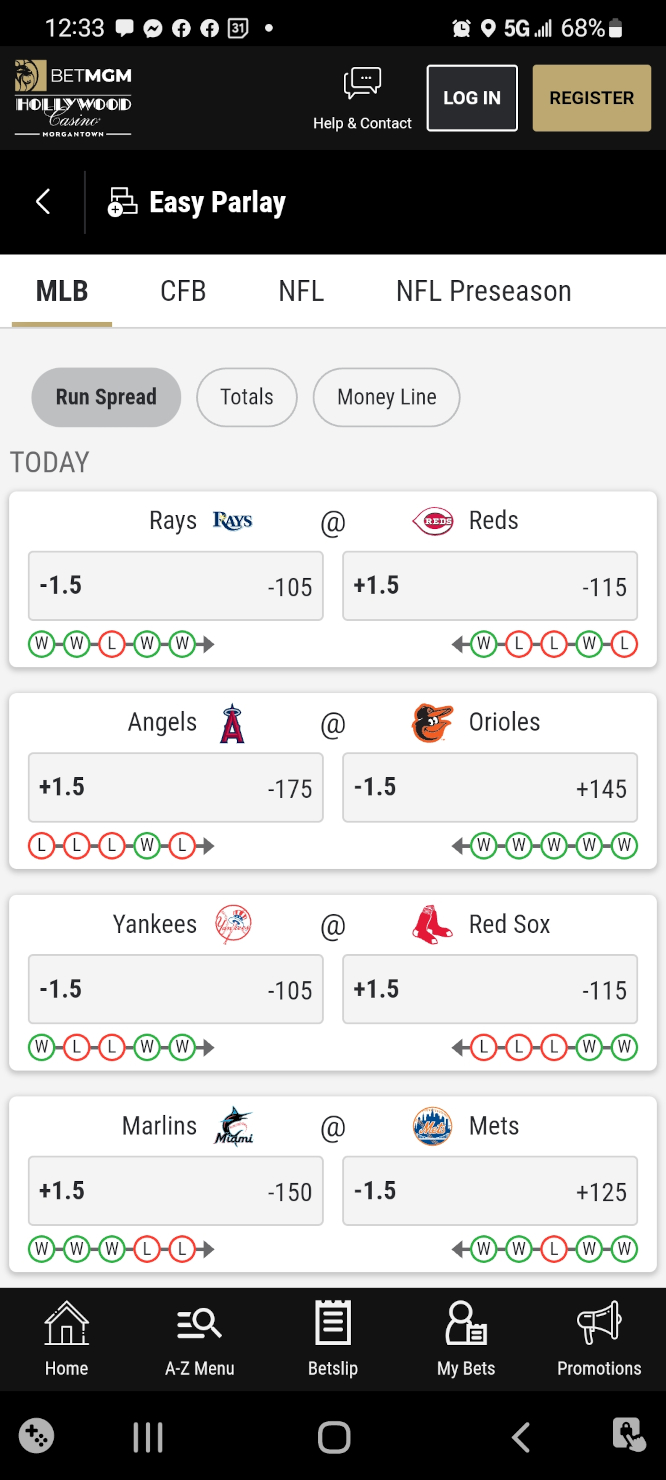Screenshot of a mobile phone displaying an online sports betting website interface. At the top of the screen, the status bar is visible showing the time (12:33), active notifications for text messages, two Facebook alerts, a calendar notification, GPS status, 5G connectivity, cellular signal strength, with a battery at 68% next to a half-full indicator.

The main content area of the screenshot highlights an MGM Resorts online betting platform. On the left side, a black "Login" button in white text and a brown "Register" button are visible. Below these buttons is an "Easy Parlay" option.

Featured prominently are sections for various sports: "MLB" (Major League Baseball) in bold, underlined gray text, "CFB" (College Football), "NFL" (National Football League), and "NFL Preseason". Betting options such as spread, totals, and money line are shown for specific games: Braves vs. Braves, Angels vs. Orioles, Yankees vs. Red Sox, and Mariners vs. Mets. The betting lines include various pluses and minuses indicative of odds and potential payouts.

At the bottom is a black navigation bar with white text, listing options such as home, A to Z menu, bet slip, my bets, and promotions. Various icons, including three horizontal lines (menu icon), a square, an arrow pointing left, and a lock, are displayed at the footer.

The caption closes with a humorous tribute to Macho Man Randy Savage, known for his wrestling persona, adding a light-hearted touch to the otherwise technical description.